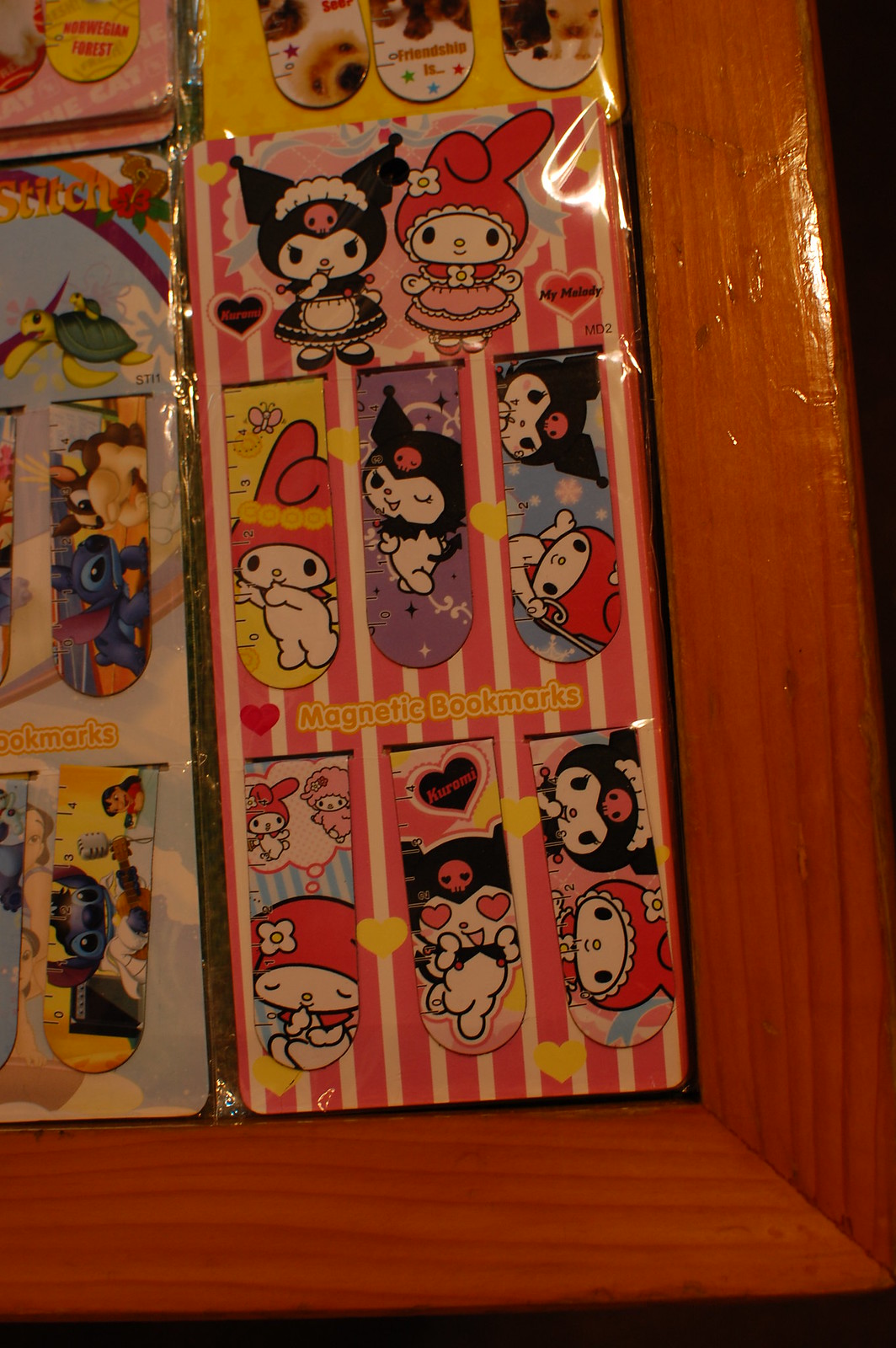The image depicts a medium reddish-brown wooden frame, partially visible at the bottom and one side, meeting at a corner. Inside the frame are several packets geared towards children, protected by clear plastic packaging. Prominently displayed are two rows of magnetic bookmarks, featuring a variety of characters. Among them is Hello Kitty, dressed in different outfits, and other manga-like designs, including characters with black dresses, pink dresses, and a blue animal with a small green turtle on its back. The packaging has "magnetic bookmarks" written in bold yellow and orange print. The entire setup appears to be placed on a wooden surface.